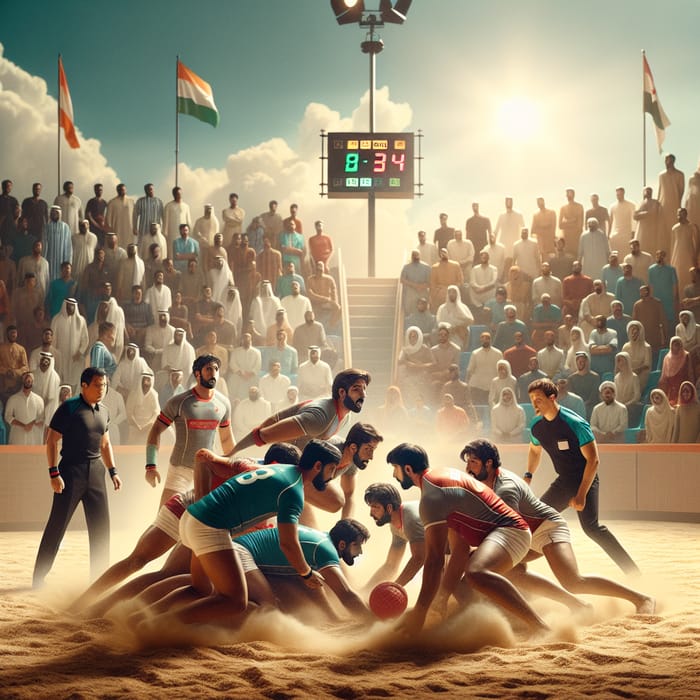This intricate painting depicts an intense sporting event taking place in a circular, sandy pit. At the heart of the scene are two teams of men grappling for a red ball, suggesting a vigorous game possibly reminiscent of rugby. Each team has distinct uniforms: one team wears turquoise shirts and white shorts, while the opposing team sports gray shirts with red accents and white shorts. All the players are barefoot, uniformly featuring brown hair, beards, and mustaches, adding to a sense of unity and tradition.

Flanking the players are two referees dressed differently—one entirely in black, and the other in black pants with a black and turquoise shirt, both closely monitoring the action. Surrounding the pit, a large audience, predominantly in traditional Arabic attire, watches intently from the stands. Most spectators wear white robes and headscarves, although some are bareheaded and in different colors. 

Above the captivated spectators is a prominent scoreboard displaying the figures 8 and 34, with the 8 in green and the 34 in red, accompanied by big lights and flanked by three flags: one with orange, white, and orange stripes; the second with orange, white, and green stripes; and the third with red, white, and black stripes. The background showcases a beautiful blue sky adorned with large, fluffy clouds, further adding to the dynamic and captivating atmosphere of the painting.